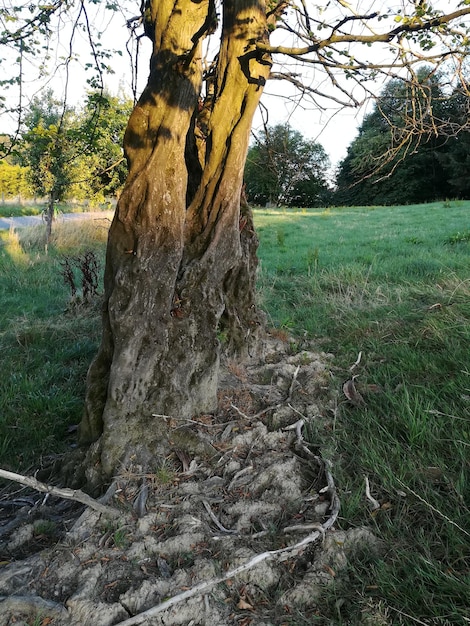A knotty tree stands prominently in an outdoor setting, its gnarled roots creating an intriguing network at its base that seems to repel grass growth. Surrounding the tree, lush green grass stretches out, contrasting with the barren ground immediately around the roots. The tree itself has sparse branches adorned with a few small green leaves, indicating the arrival of spring. In the background, a collection of trees brimming with vibrant green foliage creates a backdrop that intensifies the scene’s rich greenery. The sky is predominantly gray, casting a muted light over the landscape, though occasional beams of sunlight break through. Far off in the distance, a strip of white pavement, likely a road, sneaks into the background, its bright surface standing out against the surrounding nature. Overall, the photo exudes a sense of calm daylight amid early springtime transformation.